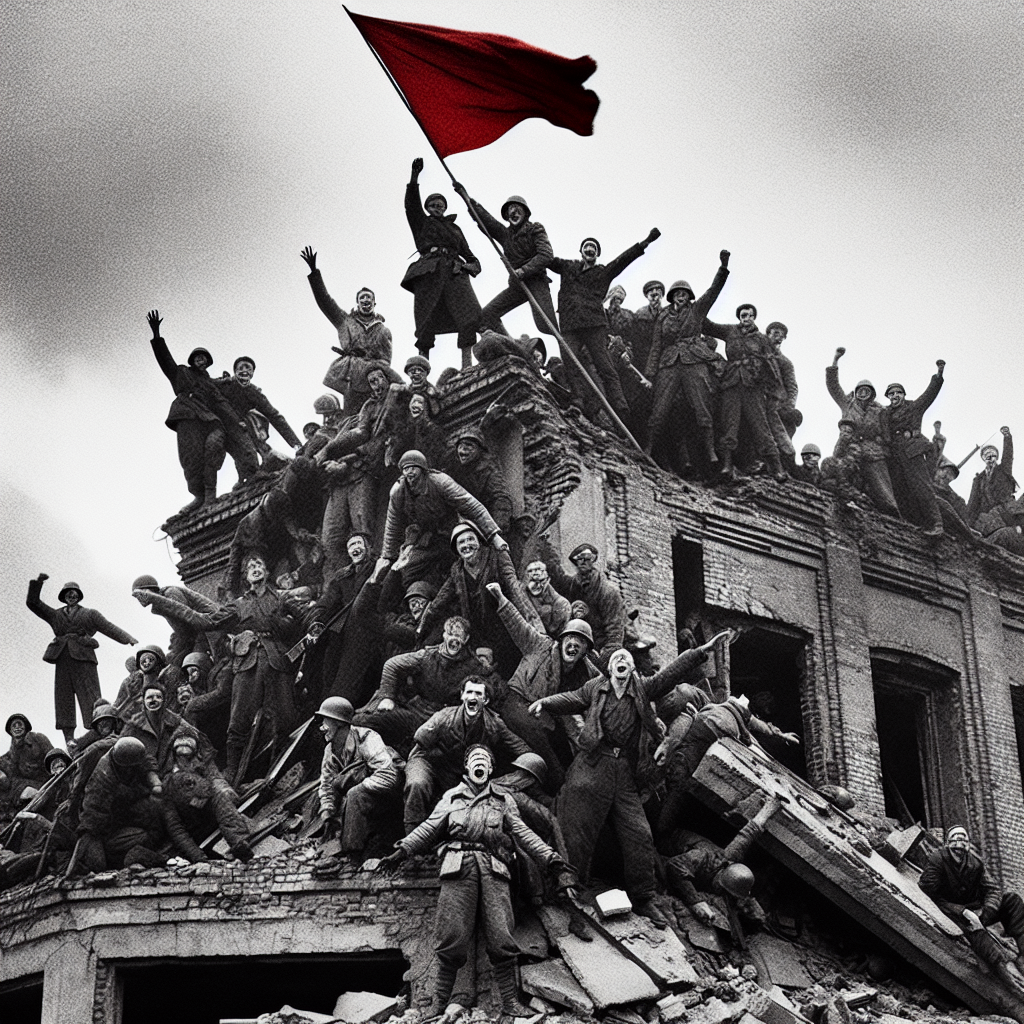This black-and-white photograph, likely historical, captures a dramatic scene on a large, partially destroyed brick building. The crumbling structure reveals both a first and second story, with the debris visually dominating the right to the center of the image. A crowd of approximately 50 to 100 men, possibly soldiers equipped with long pants, long shirts, and helmets, are standing on the roof and amidst the rubble. Notably, their faces appear severely distorted, possibly due to intentional manipulation or the men wearing masks. At the top of the building, one soldier prominently holds a large flagstaff with a vibrant red flag, the only burst of color in the otherwise monochromatic scene. The sky in the background is a pixelated grey, suggesting cloudiness. The camera angle is positioned upward, emphasizing the towering presence of the soldiers and the flag against the overcast sky.